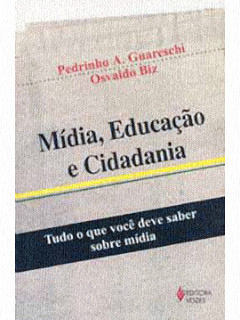The image is a grainy photograph of a book cover with a tan background. At the top of the cover, in red text, it says "Pedrino A. Guareschi" followed by "Osvaldo Biz" both tilted slightly counterclockwise. Below these names, there are blue letters reading "Mídia, Educação e Cidadania," which are horizontally aligned in the middle of the cover. Further down, a yellow stripe spans horizontally, followed by a smaller blue stripe. Below this, another section features the phrase "Tudo O Que Você Deve Saber Sobre Mídia," written in black text on a white background. Finally, at the bottom right corner, there is a small logo that is too indistinct to identify, along with additional unreadable text.